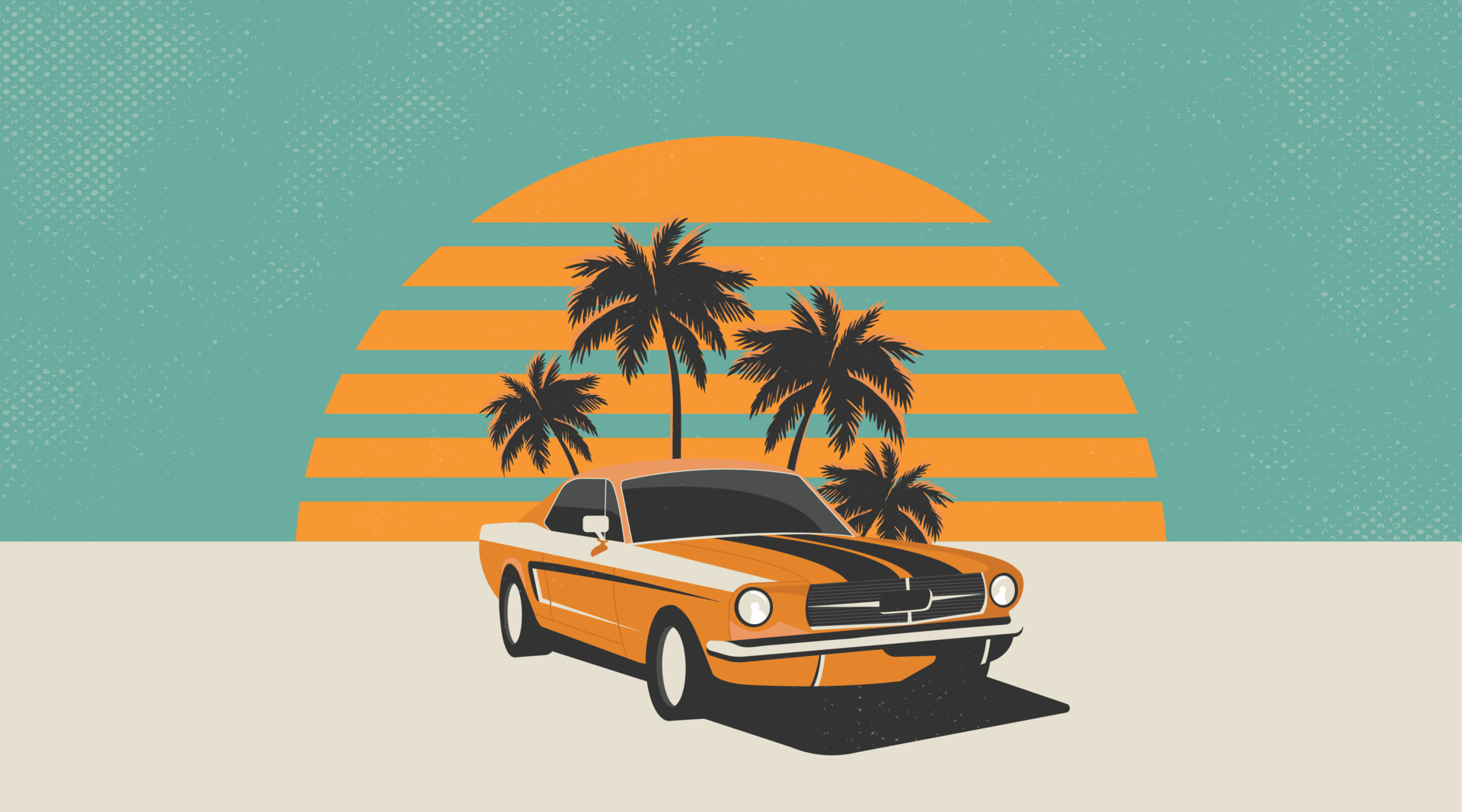This vibrant, stylized image showcases a classic 1960s muscle car, possibly a Camaro, Mustang, or Dodge Charger. The car, painted in a striking orange with two black racing stripes down the hood and some white detailing, is captured at a dramatic angle, slightly turned to the right. It sits on a sand-colored surface, casting a black shadow underneath. Behind the car, four tall, dark palm trees stand silhouetted against a unique, surreal sun. The sun, depicted with orange and aqua horizontal stripes, creates a striking visual effect by dividing the sky into sections. The sky itself boasts an aqua hue that contrasts beautifully with the sun and the black palm trees. The overall composition evokes a sense of retro-modern artistry, blending elements of nature with classic automotive design.